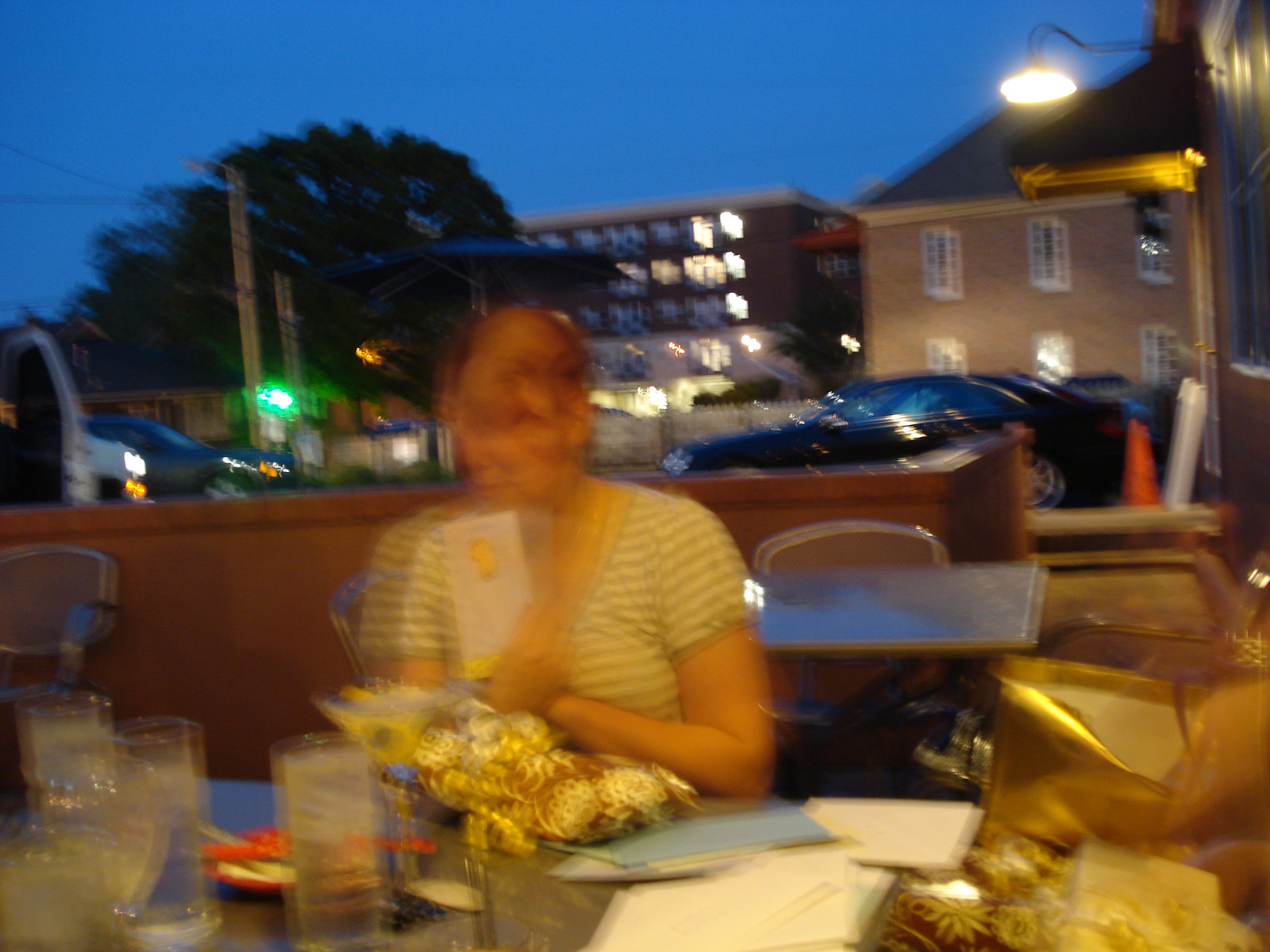In this slightly out-of-focus image capturing an urban outdoor eating area, a woman takes the center stage, exuding celebratory vibes. She is dressed in a short-sleeved, horizontally striped gold and white top. Her brown hair is neatly pulled back, revealing a joyful expression as she holds up what appears to be a birthday card, indicating she might be celebrating her special day. In front of her, a martini or margarita adds a touch of festivity to the scene, complemented by glasses of water on her left. To her right, a collection of birthday cards and presents further emphasize the celebratory mood.

The background showcases a brick wall, partially obscured by an orange traffic cone placed on the right. Behind the wall, a black car is parked, adding an urban feel to the setting. Various buildings, including a prominent brick structure and another in the center of the frame, create an architectural backdrop. A tree adds a touch of nature, its presence contrasting with the surrounding edifices. All of this is bathed in the serenity of a dark blue evening sky, adding depth and charm to the overall ambiance.